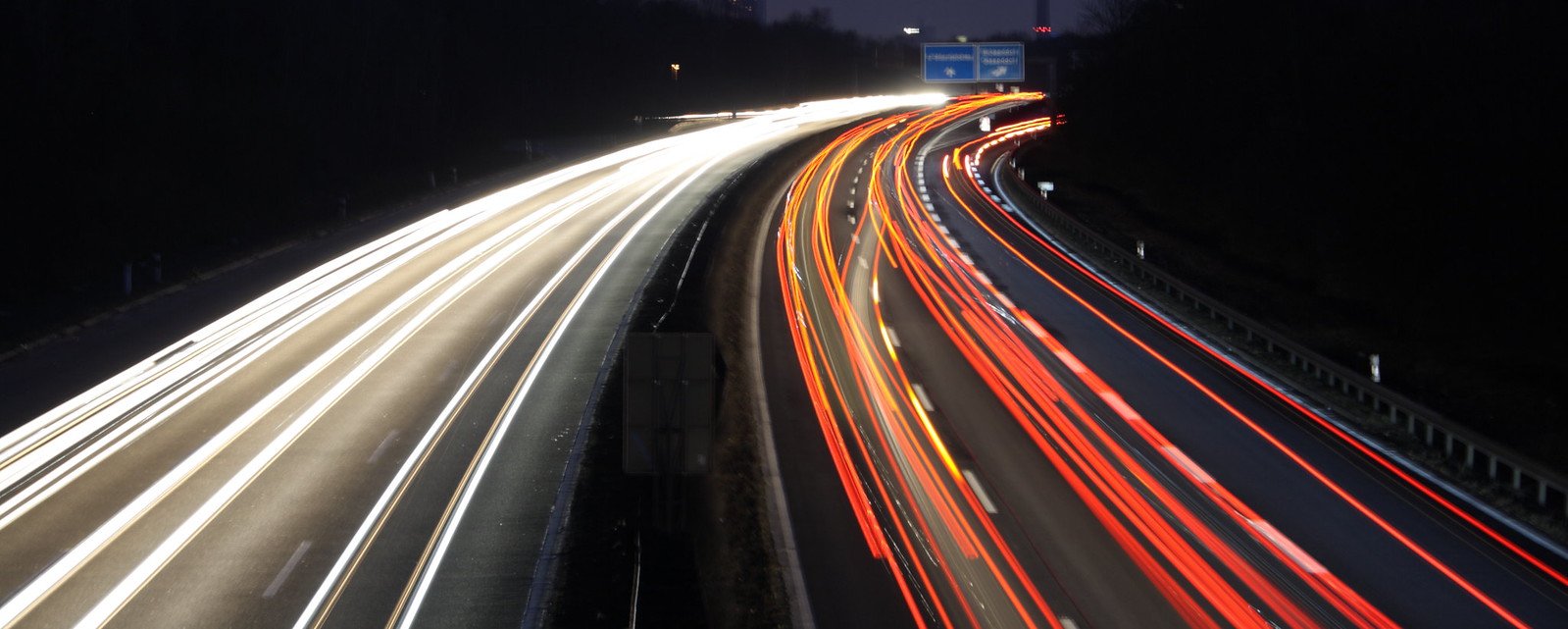The image captures a night scene of two curving highways, likely a northbound and a southbound route, intersecting at an overpass. The two roads bend towards the top right corner of the image. On each highway, streaks of lights indicate moving traffic: bright orange lights stream along the right side, likely from the taillights of cars heading north, while on the left, white lights, presumably headlights, travel south. Above the roads, a blue freeway sign with white arrows and descriptive exit information is visible. The highways are bordered by guardrails, beyond which the landscape fades into darkness, with faint outlines suggesting the presence of trees or bushes. The overall scene is dominated by the contrast between the illuminated traffic and the surrounding night, emphasizing the motion and energy of the vehicles against the stillness of the dark environment.